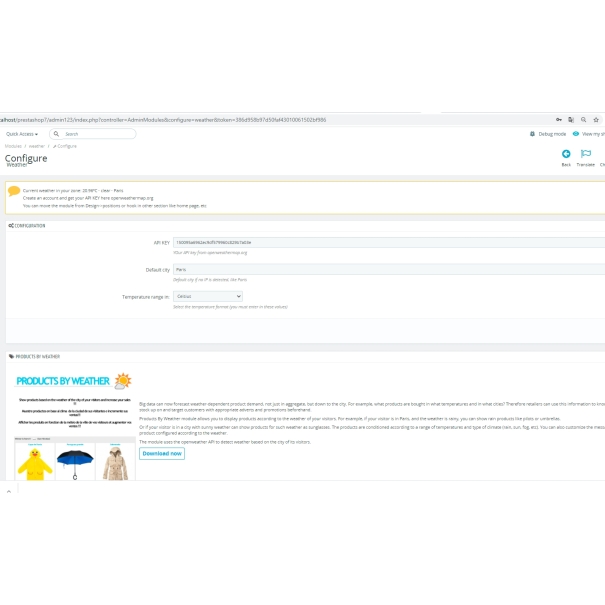Here's a cleaned-up and detailed descriptive caption for the image:

---

The web page features a standard address bar at the top, though the small font size makes it difficult to read. Below the address bar is a section labeled "Quick Access" accompanied by a search bar. This area displays three options, which are also difficult to decipher due to their small, light gray font. 

Following that, there is a heading—possibly "Configure Initiative"—with several progress bars beneath it. Adjacent to this is a speech bubble icon filled with yellow, containing three lines of text. Unfortunately, the text is in light gray on a white background, making it nearly illegible.

Further down, there is a form with multiple fields, each presumably intended for user input. These fields are also challenging to read, but the final one appears to be a drop-down menu. Each form field is accompanied by a brief explanatory note in even lighter gray text, intended to guide the user on what to enter.

At the bottom of the page, a section titled "Products by Weather" features an icon of the sun partially obscured by a cloud. This section suggests items such as a raincoat, an umbrella, and a heavy coat, possibly akin to a London Fog coat, for varying weather conditions.

---